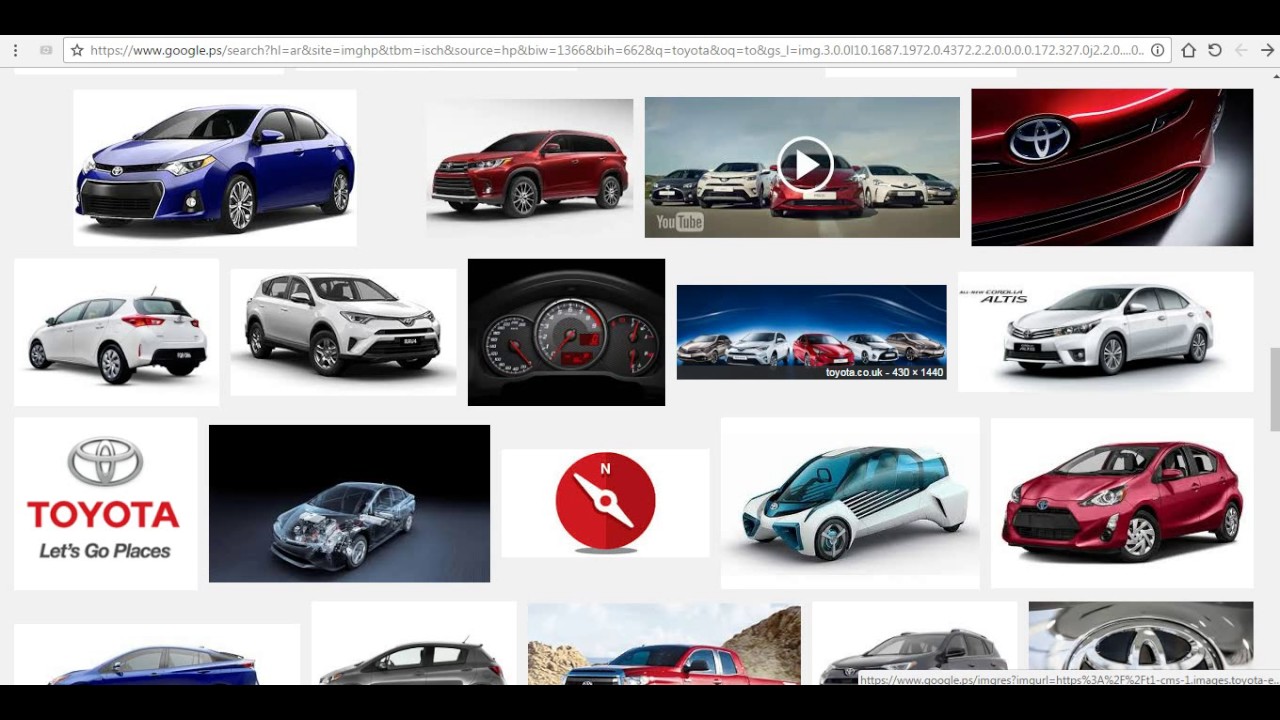This image is a detailed screenshot of a web page showcasing an array of Toyota vehicles. The layout is clean and structured, bordered at the top and bottom by thin black lines. Just beneath the top border, an address bar is visible, flanked by icons on both the left and right sides. The page is illustrated with a variety of car images, presented in a grid format.

In the bottom left corner of the webpage, the recognizable Toyota logo is prominently displayed alongside the tagline "Toyota, Let's Go Places." The top row features four distinct images: a metallic blue car, a red SUV, a YouTube video thumbnail showcasing several Toyota cars, and a close-up of a red Toyota logo on the grille of a car.

Moving to the second row, five images are displayed: a white Toyota, a white SUV, a close-up of a dashboard, an illustration depicting five cars, and another white car. The third row continues the visual journey with the Toyota logo, a prototype car, a gas gauge, a futuristic space-themed car, and a red car.

The bottom of the image partially shows five additional images which are cut off by the footer. These include, from left to right: an electric blue car, a small gray hatchback, a red truck in the center, a black truck beside it, and finally, a close-up of a silver Toyota logo in the lower right-hand corner. On the right side of the image, a thin light gray vertical scroll bar can be seen, indicating that the page can be scrolled for more content.